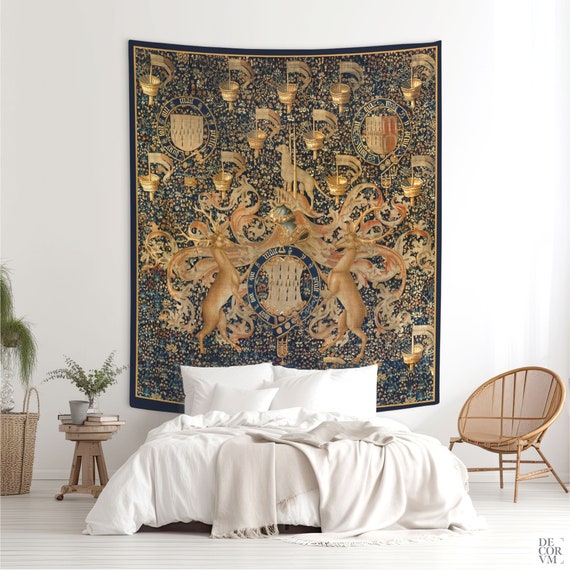The image features a bedroom with a prominently displayed bed at the bottom center, dressed in white comforters and sheets, some with tassels draping to the floor. The bed is adorned with two large white pillows. Above the bed, a large, museum-quality blue and gold tapestry from the mid-1500s to 1600s era dominates the wall, exhibiting intricate designs including two deer standing on either side of a central shield, a hunting hound above the shield, and various noble crests and flags. To the left of the bed, there is a small bedside table with a vase containing plants and several books. Additionally, a basket is also seen nearby. On the right side of the bed stands a unique circular wicker chair supported by wooden legs. The room has natural light streaming in from the right, possibly from a window out of the frame. At the bottom right of the tapestry, text reads "D-Core VM," which appears to be a logo.